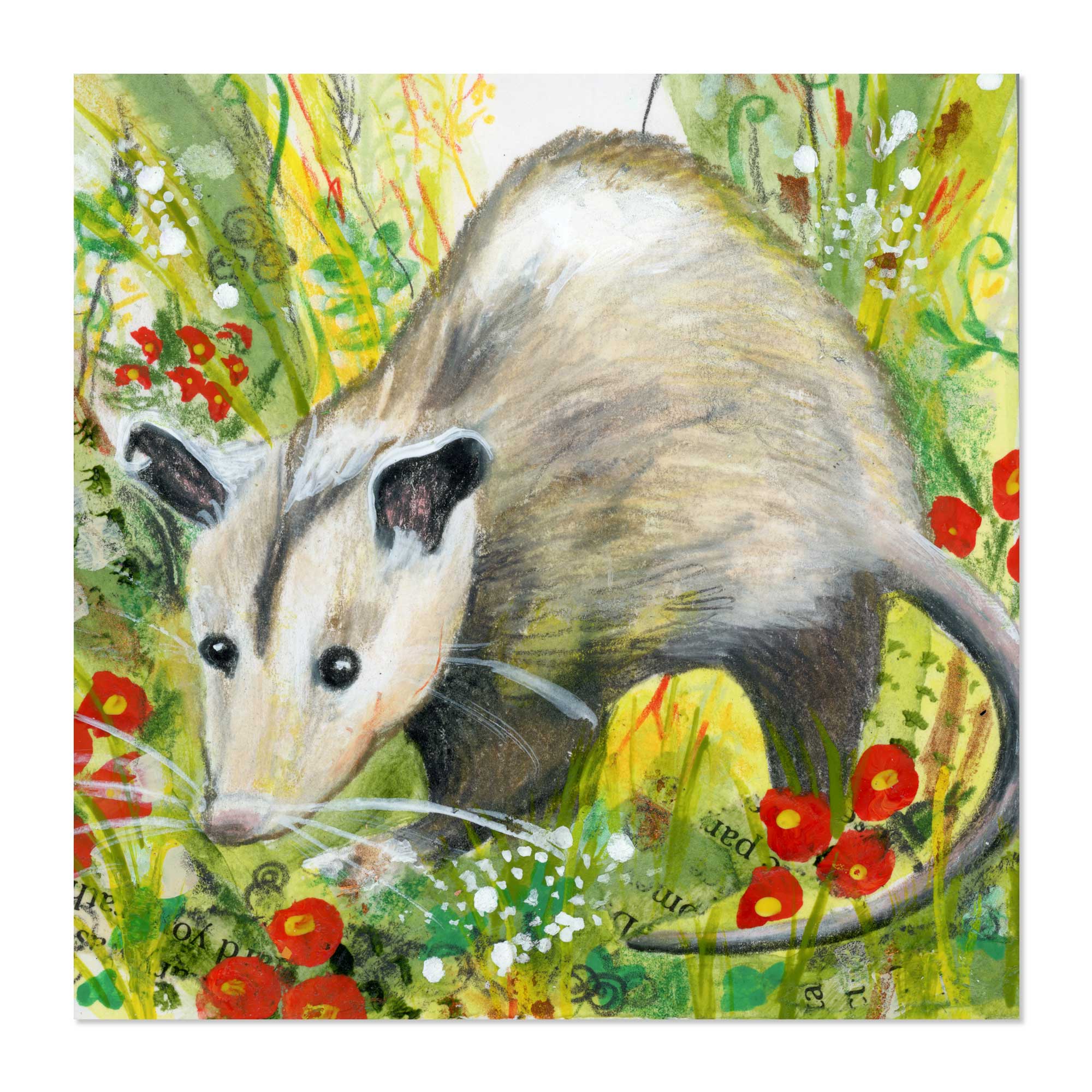The image is a detailed painting of an opossum positioned centrally amidst a lush, tall weeded area with vibrant red and yellow flowers. The opossum features a distinct white face with a black stripe across its forehead, black eyes, black ears, and a predominantly grayish body that transitions to white at the top. Surrounding the opossum, the greenery includes swirling patterns of green and yellow leaves and red circular flowers with red centers, enhancing the vividness of the scene. The background is hinted to contain pieces of newspaper parchment, adding texture and depth. White specks of paint are scattered above the possum, particularly toward the top corners, contributing to the intricate artistry. The lower part of the painting includes dark printed text, prominently decorating the bottom side.